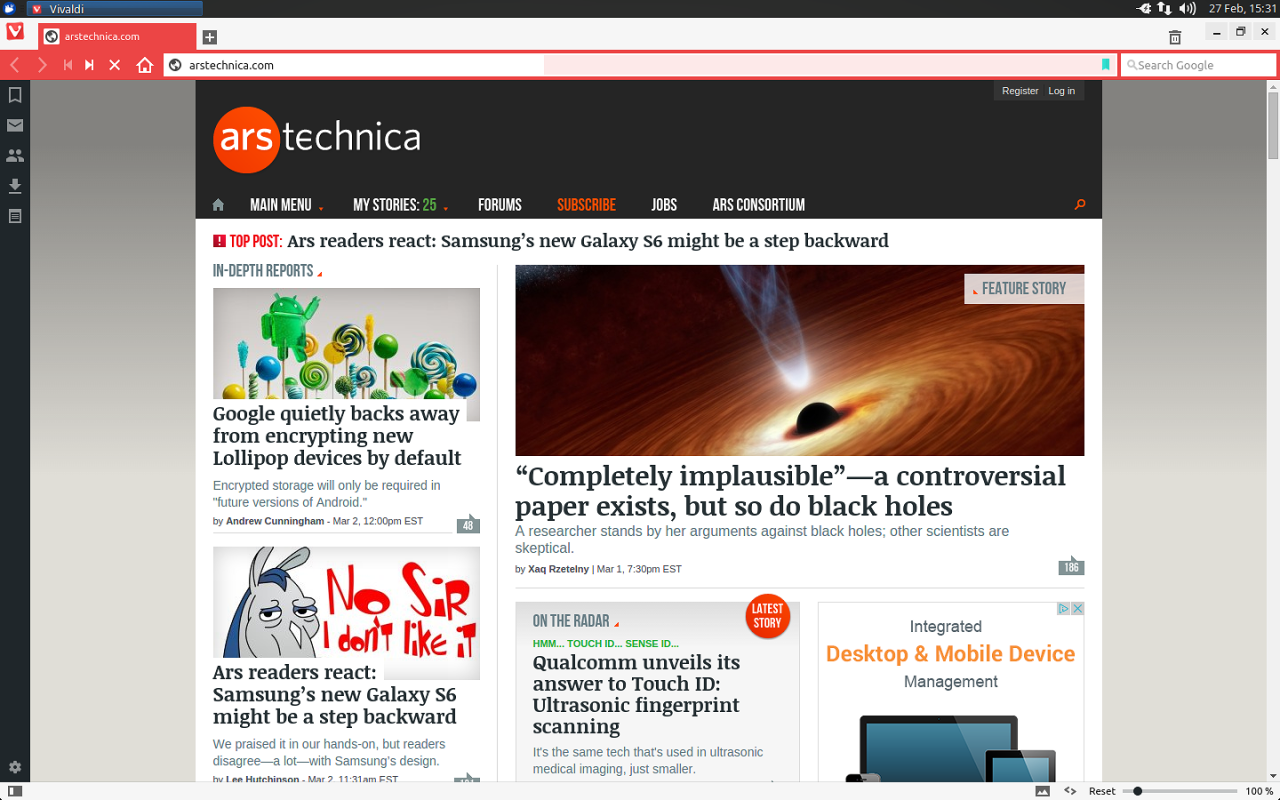This is a detailed screenshot from a website. The top border of the image is a thin black line. In the top left corner, there is a blue circle containing a white emblem. Next to it is a blue search bar with a red square that has a white "V" inside. To the right of the search bar, "V-I-V-A-L-D-I" is written in white letters. On the right side of the top bar, the time is displayed as "1531" in white, followed by "27FEB" and a full volume sound icon. Next to the sound icon are white arrows pointing up and down.

Below this, there is a gray border. On the right side of this border, there are a series of icons: a black "X," a black square, a black dash, and a delete icon. Farther to the right, there's another red square with a white "V" and a small red pop-up tab displaying a white square with a black globe icon. The text on the tab reads "A-R-S-T-E-C-H-I-N-C-A dot com." Outside this tab, there's a small black square with a white plus sign.

Beneath this section, on the left side, a black border runs down with five clip-ons. Following this is a two-inch gray border on both the left and right sides.

The central part of the image resembles a homepage. The top inch is a black border. In the center, there's a large orange circle containing "A-R-S" in white, with the word "Technica" written outside of it. Below this logo are six drop-down tabs; the first three are in white, the fourth one has orange lettering, and the last two are white. Under these tabs, there are images and clickable articles.